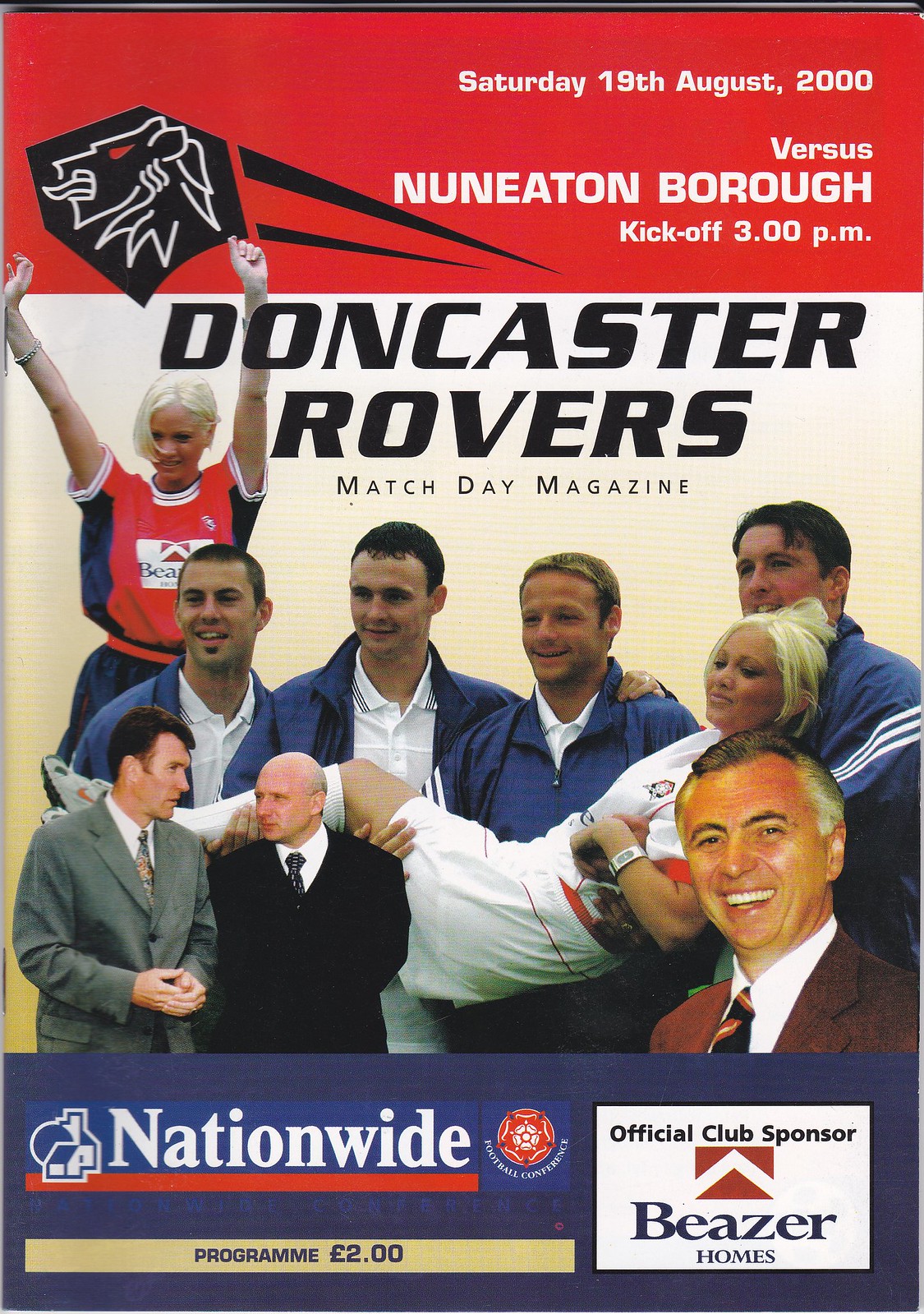The cover of the Doncaster Rovers Match Day Magazine, for the match against Nuneaton Borough on Saturday, 19th August 2000, features a vibrant and dynamic layout divided into three distinct sections. Center stage is a striking image of four men dressed in blue blazers and white undershirts, lifting a blonde female player in a white uniform who is laid across their arms. The top left corner showcases another blonde female soccer player with her arms raised in a celebratory pose. Situated in the bottom sections, the cover includes two men in suits on the left, presumably the team coaches, and another suited man on the right, the trio adding a formal touch to the overall energetic theme. Enhancing the visual composition, the top section features a red rectangular box with white lettering detailing the match date, opponent, and kickoff time. The team logo, a white lion on a black background, is prominently displayed below the text. The bottom segment is designed in blue, highlighting sponsor logos including Nationwide and Beezer Homes, with a boxed note indicating the program price of £2.